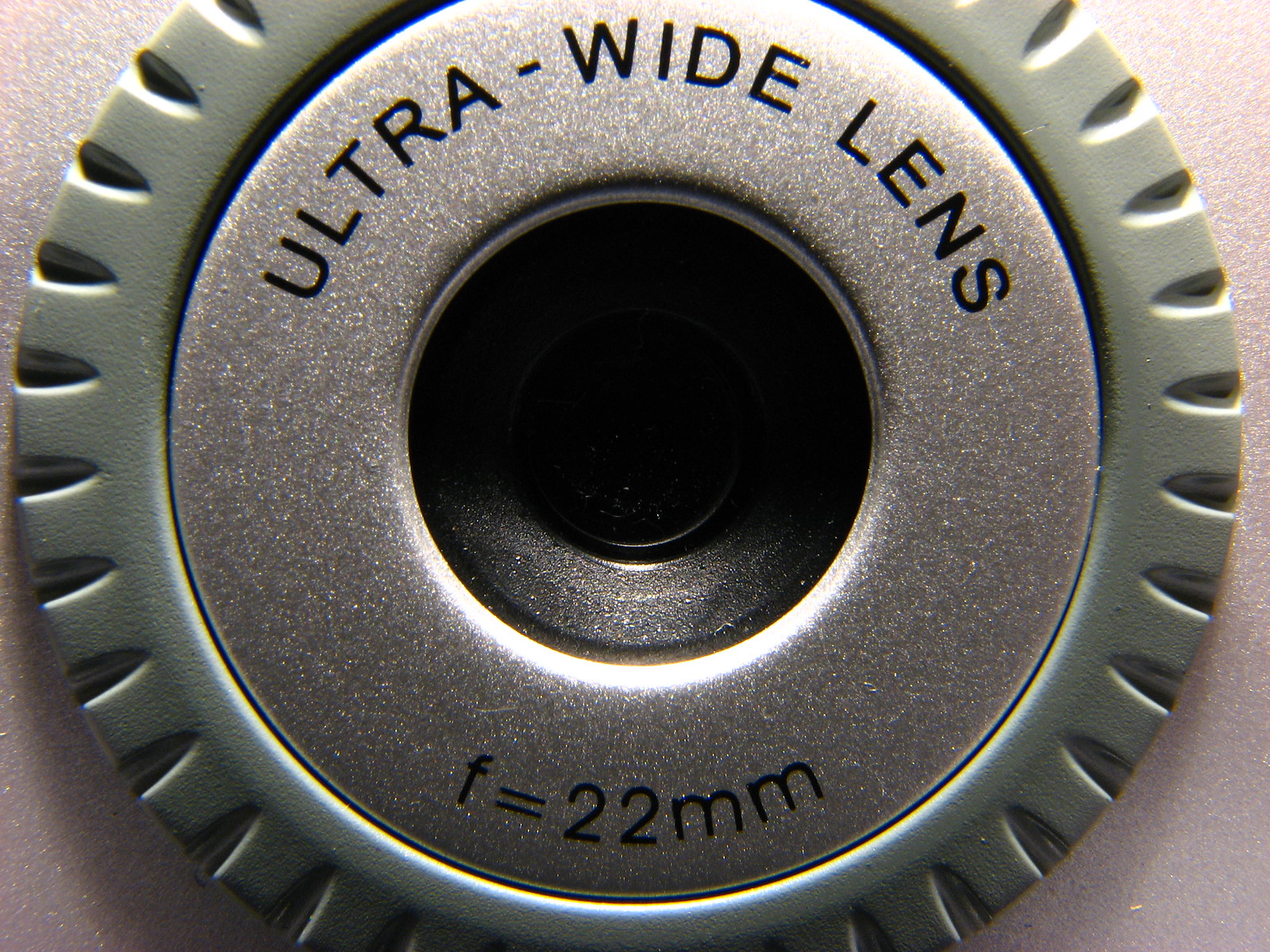The image is a high-quality, close-up color photograph of a camera lens. The lens dominates the entire frame, showcasing intricate details and clarity. The camera itself appears silver or gray, possibly made of stainless steel. The central part of the lens is black, likely plastic, encasing the glass lens. Surrounding the black center, there is a silver ring with embedded sparkly bits. This ring is inscribed with "ultra-wide lens" at the top and "F = 22 mm" at the bottom. Encircling the silver ring is a green protector with notches, adding a textured border. The background remains silvery and sparkly, enhancing the focus on the lens.